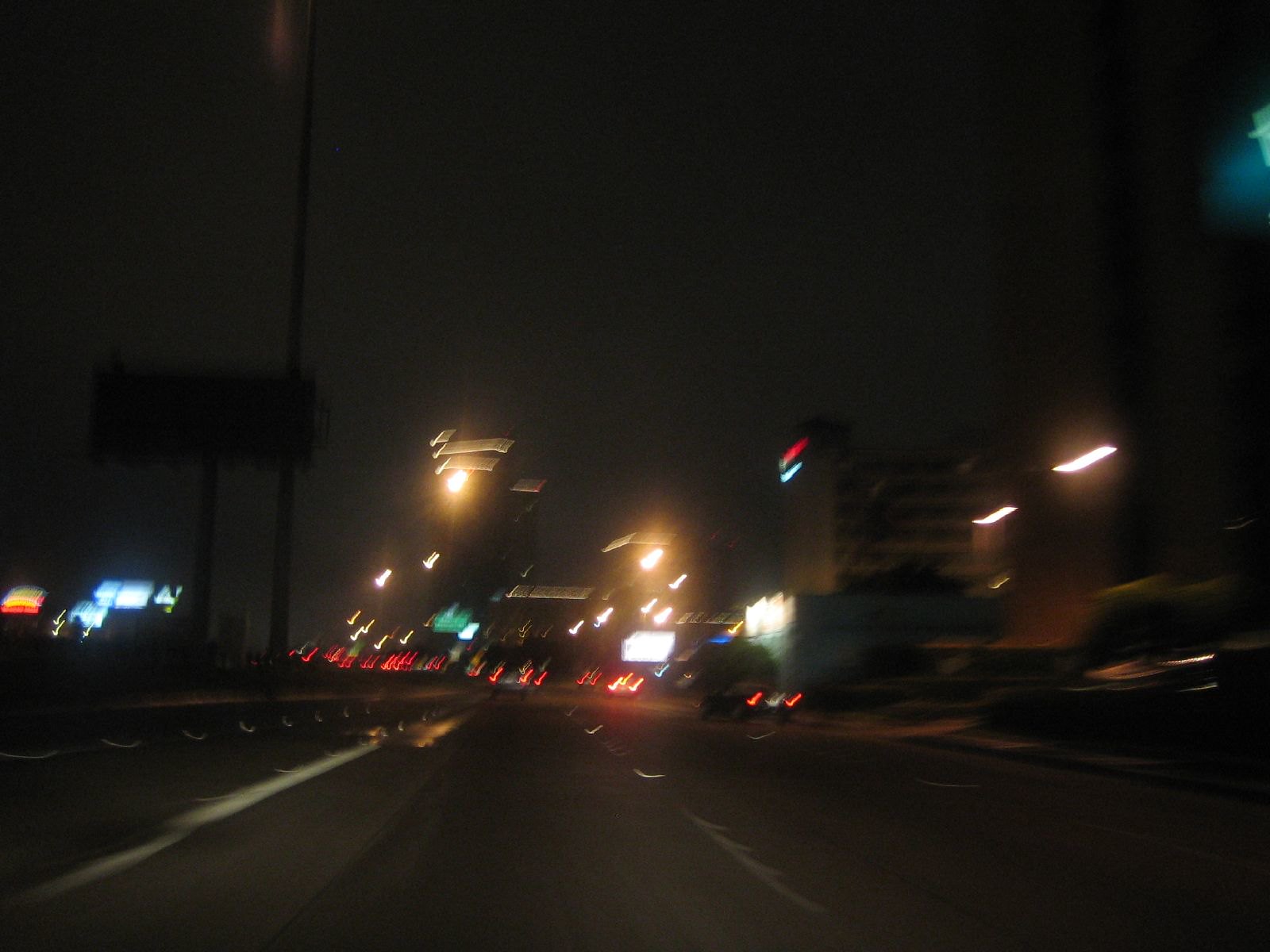A blurry nighttime photograph captures a view from a moving vehicle on a multi-lane road. The sky is a deep black, punctuated by the glow of numerous streetlights. In the distance, the silhouettes of various buildings, including a hotel and several skyscrapers, rise against the dark backdrop. The road ahead is paved with smooth black asphalt, marked with white lines and dotted lane indicators, suggesting a five-lane highway. Multiple vehicles are visible far ahead, their red taillights creating a stream of light. Green marquees and billboards are scattered in the distance, adding a splash of color to the predominantly dark scene.